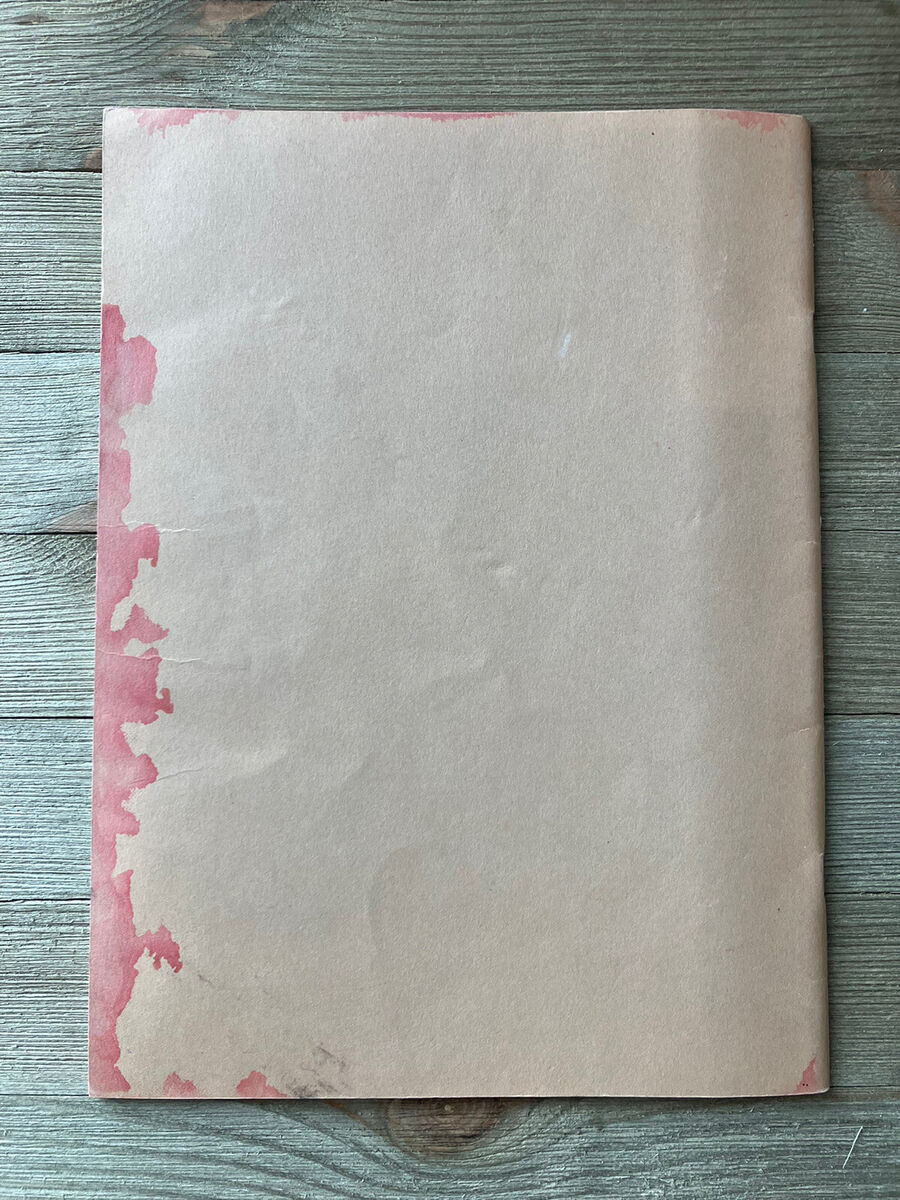The photograph depicts an aged rectangular piece of off-white parchment paper, slightly crinkled and folded on the right-hand side, resting on a wooden platform. The wooden surface is composed of seven horizontal slats, each stained a light blue color with visible brown knots and grains, especially noticeable at the top and bottom edges. The paper has pink and red watercolor blotches scattered along the top, left side, and at the bottom, adding an artistic element to its weathered texture. The scene is illuminated by natural light coming from the left, casting a soft, authentic glow over the wooden tabletop, emphasizing the distinct gray-green hue mixed with natural wood tones.